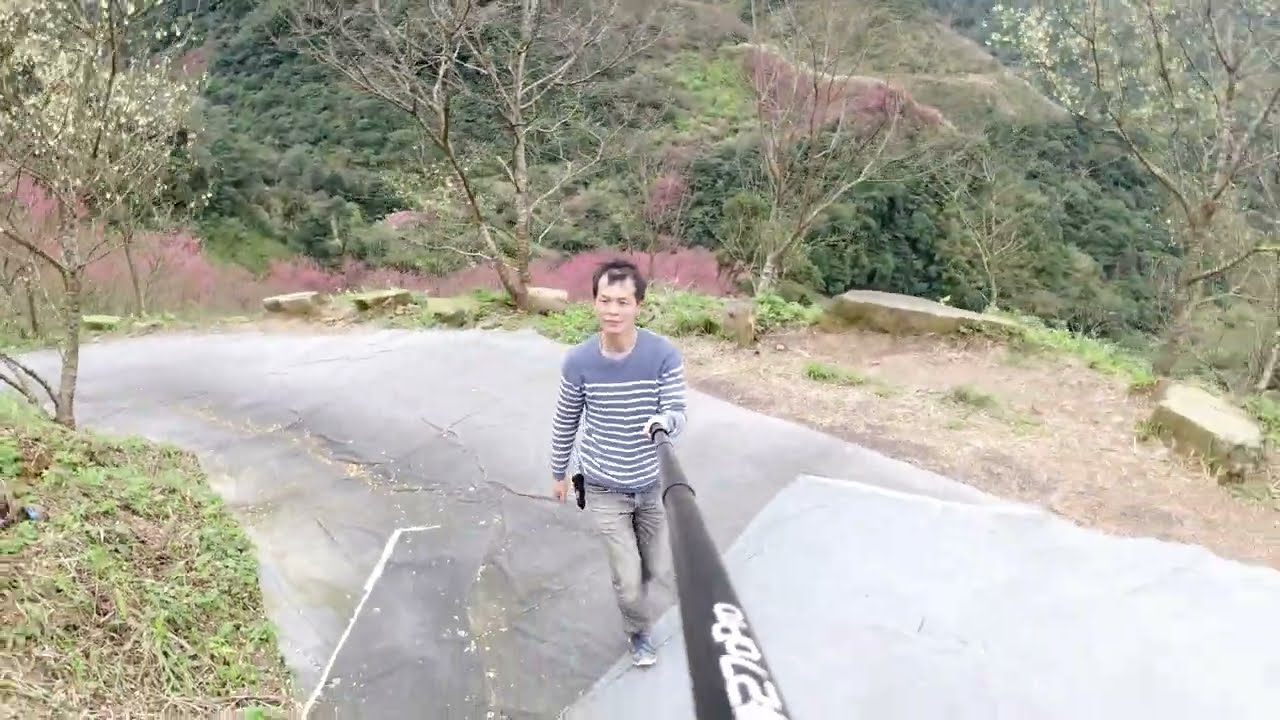The image features an older Asian man with short black hair, fair skin, and thin short black hair, taking a selfie with an extended black selfie stick, which appears prominently coming out of the image. He is centered in the picture, wearing a blue and white striped long-sleeved shirt and gray jeans. He stands on a paved trail with patches of concrete and surrounding areas of grass; some of the grass is brown and dead, while other parts are light green and thriving. Behind him, there are various trees displaying different shades of pink, light green, and dark green. The backdrop also includes a hillside covered with abundant green shrubbery, grass, and trees. The scene is bright and clear, indicating it is daytime. The overall feeling of the image is that of a casual, nature-filled walk being documented through the selfie stick.